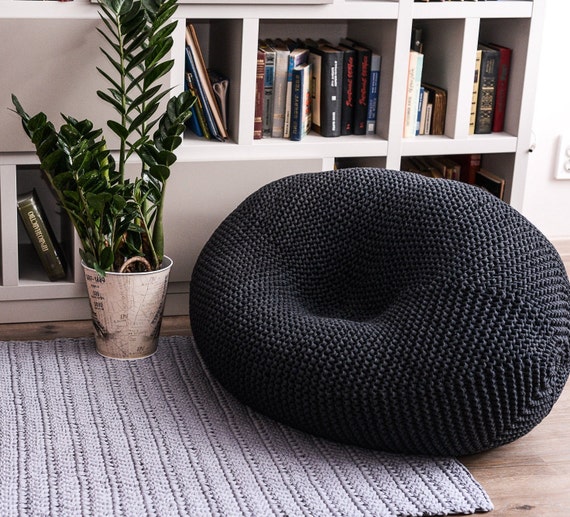The image depicts a cozy sitting nook in a living room characterized by a mix of modern and rustic elements. Dominating the foreground is a large, black, quilted beanbag chair with a noticeable indentation in the center, indicating frequent use. The beanbag rests atop a textured rug, described variously as gray or light blue with a quilty pattern. The hardwood floor beneath the rug adds a warm, natural touch to the space.

To the left of the beanbag is an old-fashioned metal bucket with side handles, serving as a planter for a tall, green leafy plant, possibly a ficus or a fern. This plant adds a touch of nature and vibrancy to the room.

Behind the beanbag is a prominent white bookcase with multiple cubby holes of varying sizes, each filled with a diverse collection of books. The design of the bookcase, with its small compartments, adds an organized yet eclectic touch to the space. On the right side of the back wall, adjacent to the bookcase, there's an electrical outlet, subtly blending into the white wall.

Overall, the scene exudes a comfortable and inviting atmosphere, perfect for reading or relaxing.